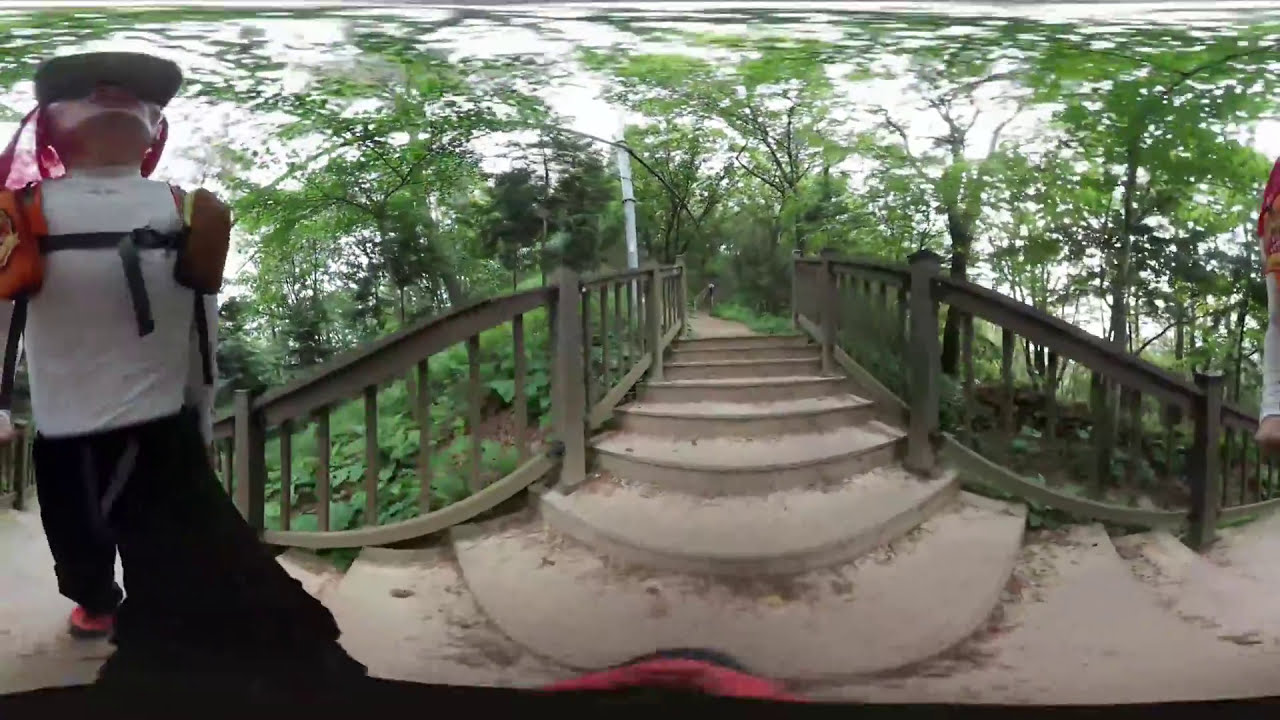This horizontal rectangular image captures a surreal and intriguing outdoor scene, taken with an unusual lens that distorts the landscape. The main focus is a walkway that begins with concrete steps, ascending to the height of what appears to be a bridge. This bridge-like path continues into the distance, flanked on both sides by wooden railings in a brownish or olive green hue. The steps and pathway are a consistent gray color, creating a stark contrast against the natural surroundings.

On either side of the walkway, dense trees stretch skyward, their forms altered into unusual shapes by the lens distortion. The foliage introduces vibrant greens into the image, while the sky above is a blank, white expanse, enhancing the otherworldly atmosphere. To the left of the walkway, there stands a figure, which distinguishes itself amid the natural setting. This figure, possibly a person or a mannequin, wears a white shirt and a hat with a pink bandana. It also sports black pants and red shoes, and appears to have an orange and black backpack. The figure's head is particularly noteworthy, as it is either obscured by a peculiar hat or resembles a frog's head, adding to the enigmatic nature of the scene.

The combination of the distorted trees, the solitary, oddly-dressed figure, and the continuous path leading into the unknown, lends the image a dreamlike, almost surreal quality, pulling viewers into a curious and contemplative state.